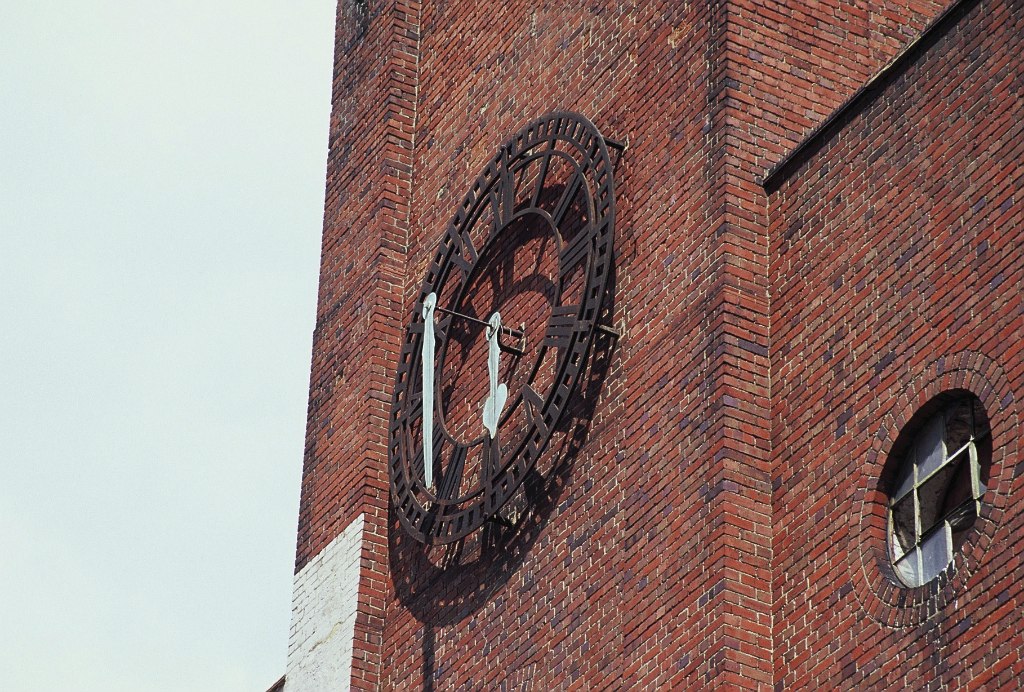In this photograph, the side of a large red brick building dominates the scene. The focal point is a substantial, round metal clock affixed to the building's wall, showcasing Roman numerals integrated seamlessly into its metallic frame. The clock features two white hands, although their exact positions are obscured due to the angle from which the image is taken. Located on the bottom left of the clock, there is a small section of the brick that has been spray painted white. On the bottom right corner of the image, a circular window framed with bricks is visible, adding to the architectural character of the building. The left side of the image reveals an expanse of white, hazy sky, indicating an overcast day.